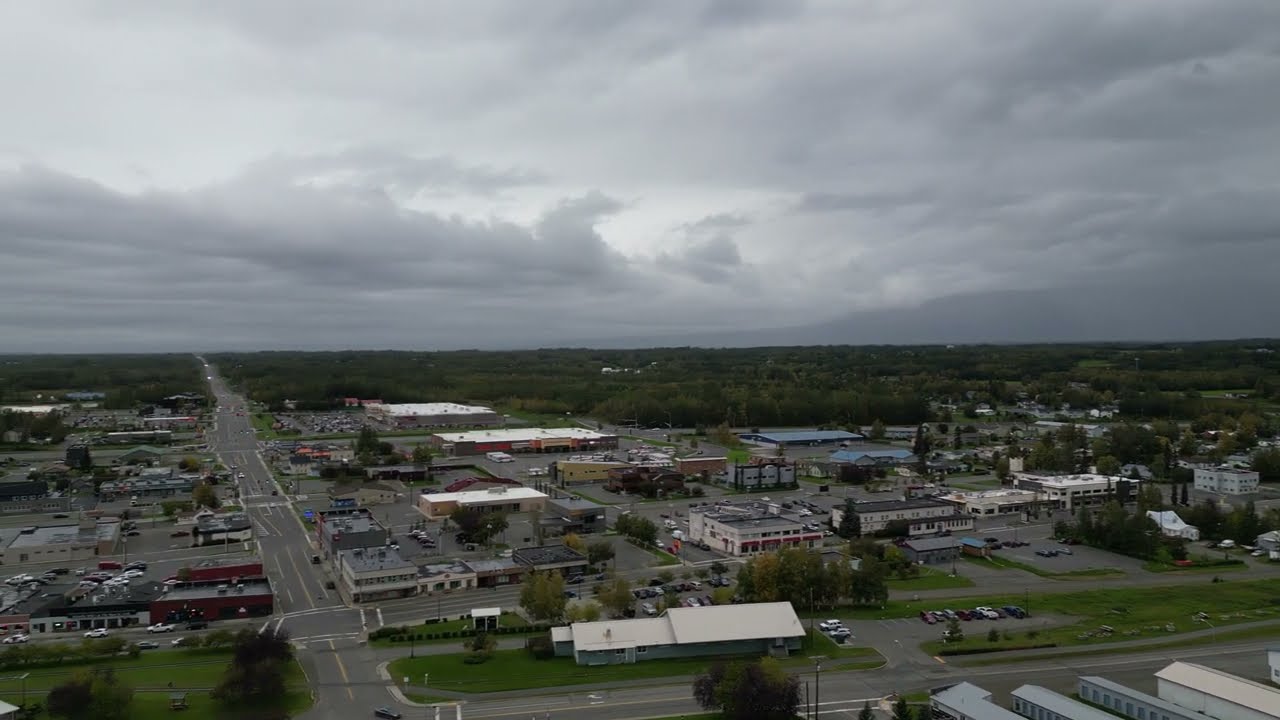This overhead photograph, captured from a high perspective, presents a small town or suburban area on a heavily overcast day. The top half of the image is dominated by a dark, cloudy sky, suggesting an impending storm. There’s a hint of light breaking through on the left side, but the overall ambiance is gray and somber. Below the skyline, the town is sprawling with short, low-rise buildings that likely include office buildings, small commercial establishments, and possibly a mini mall, indicating a business district. 

Prominent roadways traverse the town, with a four-lane road running vertically down the left-hand side and multiple cross streets cutting across horizontally. Despite the detailed network of roads, there are remarkably few cars seen traveling. The greenery of the area is evident, with patches of grass and an abundance of trees surrounding the buildings and extending into the distance, hinting at a wooded area beyond. Additionally, expansive parking lots with numerous parked cars hint at active commercial zones. The lower half of the image contrasts with the dark sky above, as lush greens and the orderly layout of the town paint a picture of a small, quiet community with a moderate population.